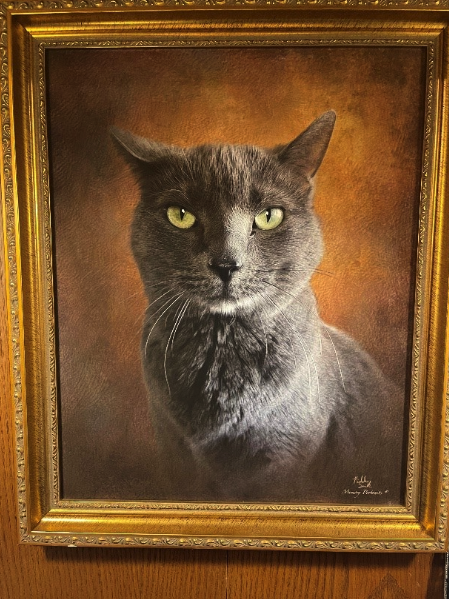The image depicts a highly realistic, framed painting of a gray cat with striking, light greenish-yellow eyes, staring directly at the viewer. The cat has a short, smooth coat with a distinctive black-tipped nose and a touch of white around its nose and mouth, giving it a photorealistic quality. Its left ear is perked up more than its right, adding to its lifelike demeanor. The painting is encased in an intricately carved, gold-colored frame that adds an elegant touch and is mounted on a medium-toned wooden wall. The background of the painting features a blend of Renaissance-style colors, including shades of ochre, light and dark brown, and nearly black hues, creating a warm yet dramatic atmosphere. In the lower right corner of the painting, a small, gold signature identifies the artist, although it is difficult to read due to its size. This exquisite portrayal of the cat, with its nuanced details and rich colors, offers a captivating view that seems almost tangible, inviting the viewer to appreciate the fine craftsmanship and lifelike representation.